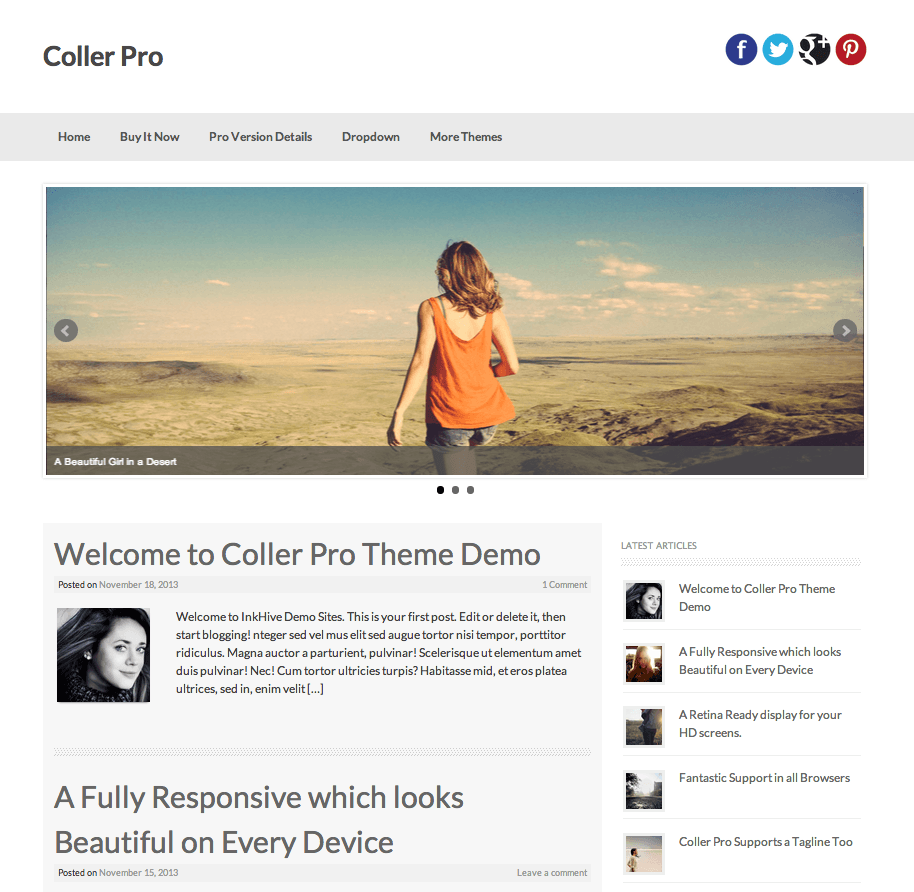The screenshot depicts a demo website for CollarPro, titled "Welcome to CollarPro Theme Demo." At the top of the page, the title "CollarPro" is prominently displayed, along with a navigation menu featuring options such as Home, Buy It Now, and ProVision Details. On the right side, icons for social media platforms like Facebook, Twitter, Google+, and Pinterest are visible.

Central to the page is an image slide featuring a striking photograph of a girl standing in a desert landscape, dressed in an orange shirt and with reddish-brown hair. The desert backdrop is characterized by brown hues, adding contrast to the girl's appearance. This image is just one in a series of three slides, but it is the only visible one in the screenshot.

Beneath the image, the page welcomes viewers with the text, "Welcome to CollarPro Theme Demo." Additional content includes placeholder text in Latin, indicating an example layout for articles which are part of the demo site. The webpage also highlights features of the theme, such as its fully responsive design, compatibility across devices, and HD screen readiness. On the right side of the page, there is an article menu listing five articles, emphasizing the blog aspect of the theme. The date displayed is November 18, 2013.